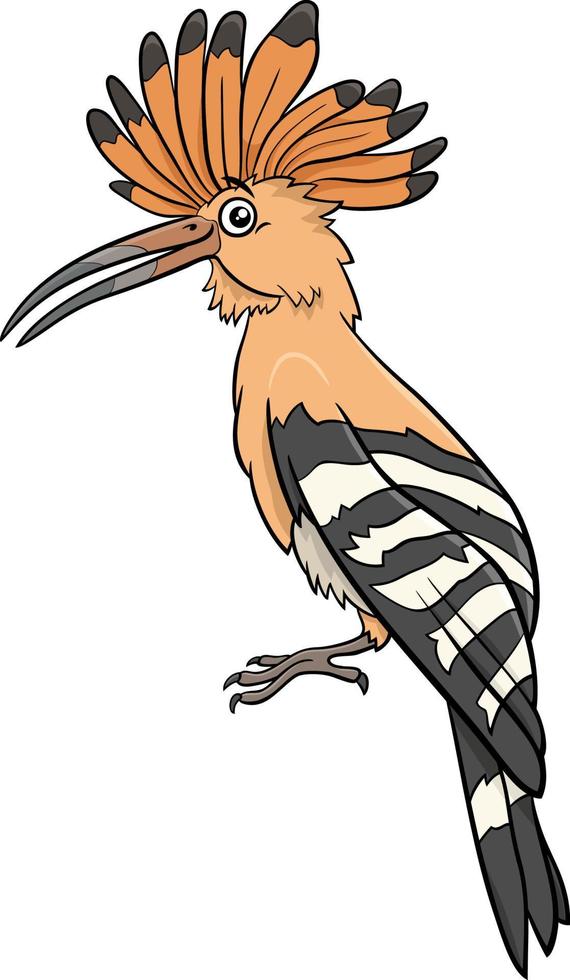This is a detailed cartoon illustration of a large bird, shown in profile facing left. The bird is predominantly orange, with a lighter orange hue covering the head, chest, and shoulder area. Its elongated beak, which is about half the bird's body length, transitions from light orange at the base to a stripe of tan in the middle, and culminates in a darker gray tip. 

The bird's wings and back feature distinct dark gray and white horizontal stripes that continue down to its long tail feathers. Notably, the bird's head is adorned with a striking mohawk-like comb of feathers, predominantly orange with black tips. The bird's eyes are open, with white sclera and black pupils, giving an impression of direct engagement with the viewer.

One visible foot is positioned out in front, displaying four digits with gray claws and dark gray, sharp talons. This detailed image, possibly computer-generated, captures the bird perched on an invisible branch, blending elements of a cockatoo with unique features such as its long, multicolored beak and zebra-like striped lower body and tail feathers.